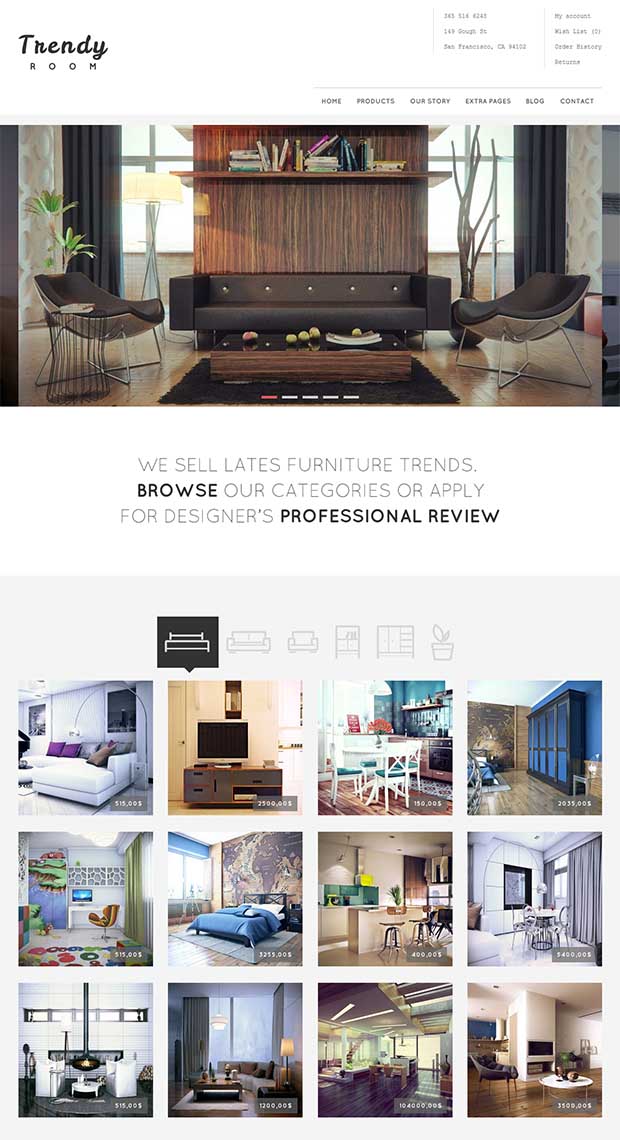This screenshot from the "Trendy Room" website features a clean, white background. In the upper left corner, the "Trendy Room" logo is displayed prominently in black font. The upper right corner offers several clickable options in gray font, though they are too small to read. Below these options, a subtle gray line separates the navigation menu, which includes links to "Home," "Products," "Our Story," "Extra Pages," "Blog," and "Contact."

The central part of the screenshot showcases an elegant yet surreal image of a living room. The room contains two uniquely shaped lounge chairs resembling half-eggs, positioned on either side of an artistically designed, seemingly uncomfortable brown couch. A brown carpet ties the furniture together. Behind the couch, a wood-grain room divider with a built-in shelf stands inexplicably in front of a window, a design choice unlikely to be practical.

Below this image, in gray font, is a promotional message: "We sell weights, furniture, trends. Browse our categories or apply for a designer's professional review."